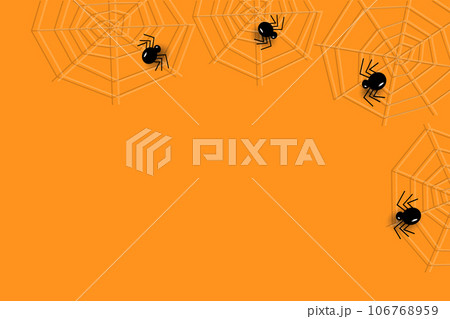The image is a digital piece of artwork with an orange background, featuring four circular white spider webs with hexagonal crossings and black spiders within them, located at the top and right side of the image. The center of the image prominently displays the word "PIXTA" (P-I-X-T-A) in white capital letters, accompanied by a 3D box symbol on its left. Extending from the corners of the image toward the "PIXTA" text are four white lines. At the bottom of the image, the text "PIXTA.jp - 106768959" is written in black, with "PIXTA.jp" denoting its Japanese origin.